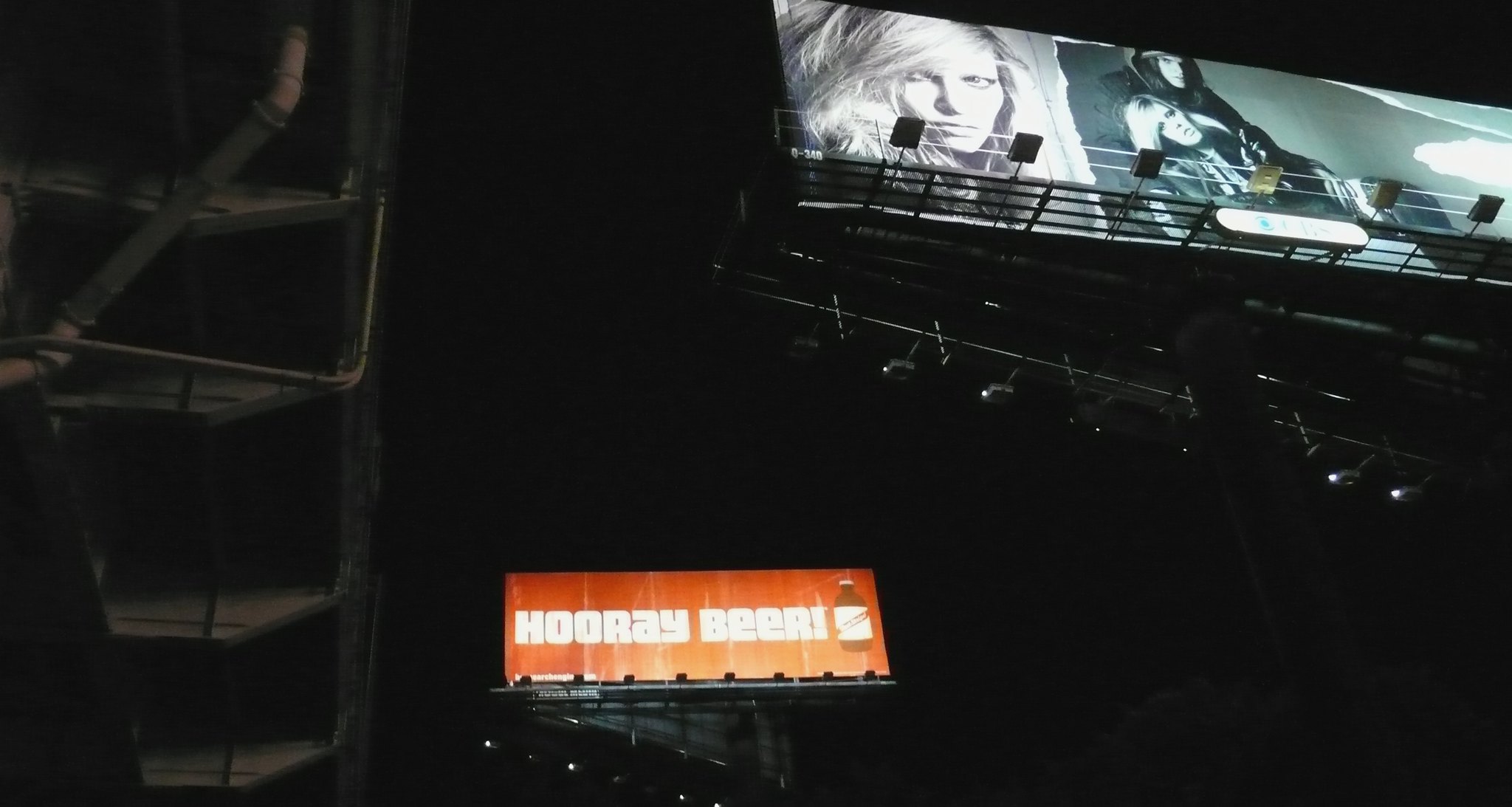In this nocturnal photograph, the inky blackness of the sky serves as a stark backdrop for an elevated scaffold that supports a prominent billboard. The left side of the billboard features a striking close-up portrait of a beautiful blonde woman with a model-like appearance. She exudes a sultry expression, highlighted by her high cheekbones and full lips. To the right of this image, another black-and-white photograph reveals the same woman in a semi-reclining pose. A man wearing a black hooded jacket stands behind her, the hood obscuring part of his face, adding an element of mystery. In the distance, a second billboard catches the eye with its vibrant orange background. Adorned with white letters, it enthusiastically exclaims "Hooray Beer!" next to an illustrated bottle of beer. The contrast between the monochrome and colored billboards creates a visually compelling scene in the silent darkness of the night.